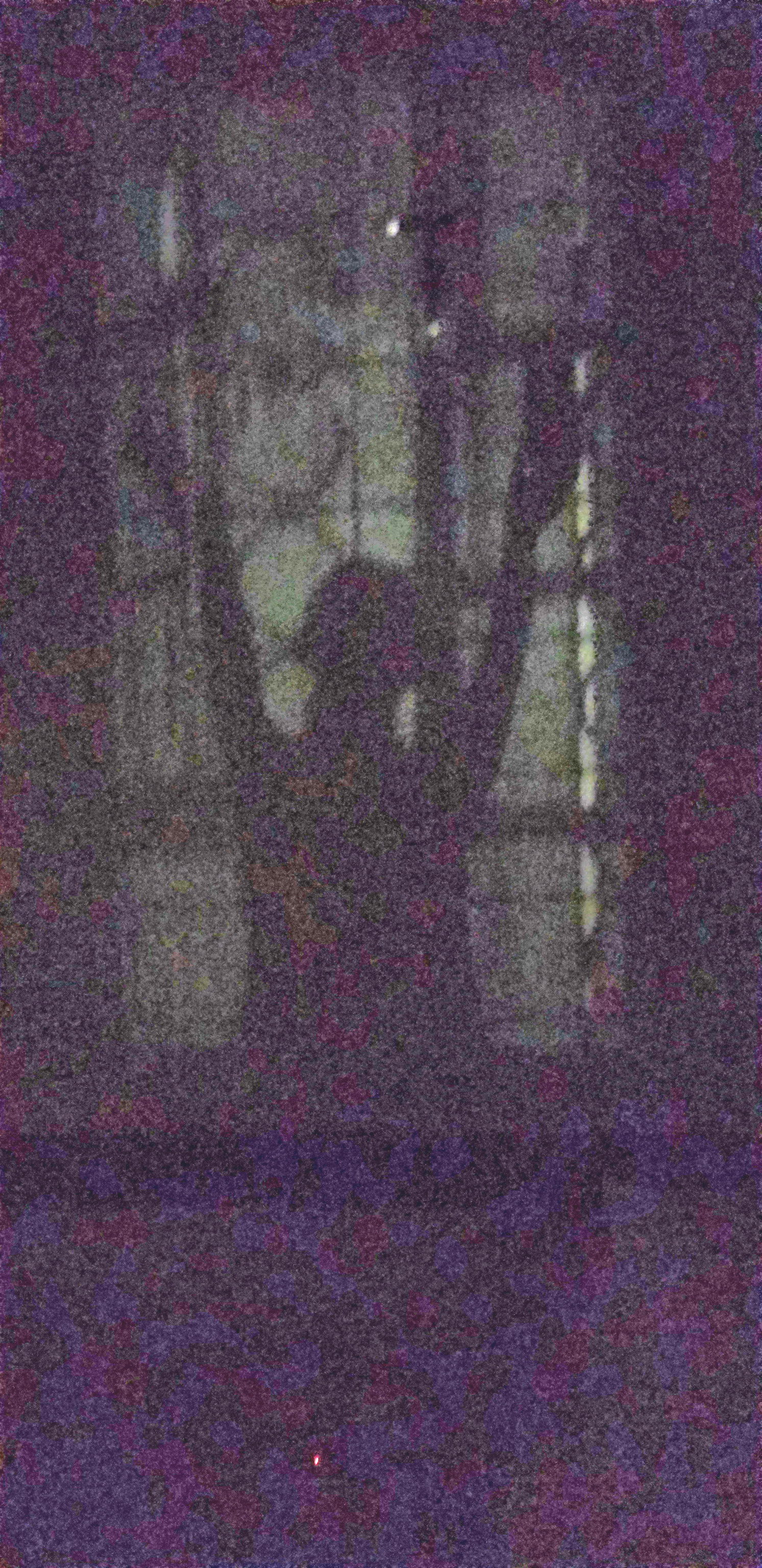In this dark, grainy photo, an indistinct silhouette of a person, possibly a woman, is captured in front of a window with thin curtains. The image's clarity is poor, filled with colored noise, including purples, blacks, reds, and a greenish-black tint, especially at the bottom where the colors fade up into the silhouette. The figure appears to be in a pose that suggests they might be sitting with their knees bent and arms upstretched towards the sky, reminiscent of a yoga posture. The room looks dark, with minimal light filtering through, perhaps hinting it is also dark outside. Faintly visible in the background are elements like leaves, trees, and maybe a fire escape, adding to the scene's shadowy and abstract ambiance.